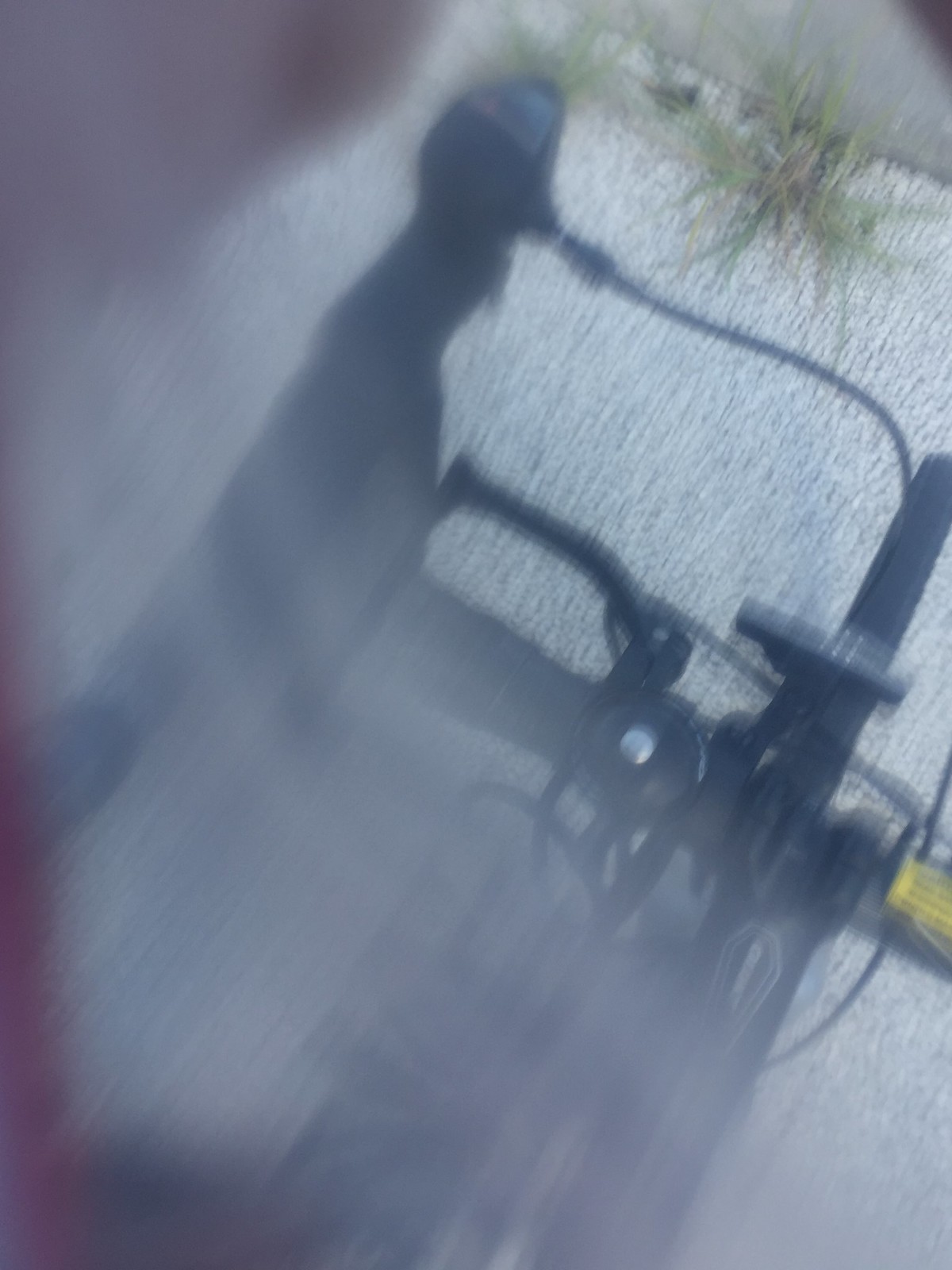The image is extremely blurry, making it difficult to decipher specific details. It appears to be taken in motion, possibly by someone riding a motorcycle or walking. The ground, which is visible, seems to be concrete with a few weeds sporadically emerging from it. A black frame dominates the lower portion of the image and could potentially be part of a bicycle. This frame features several black wires and what seems to be a handlebar. There is also a round black component accented with a hint of silver. The exact nature of the objects remains unclear due to the significant blur.